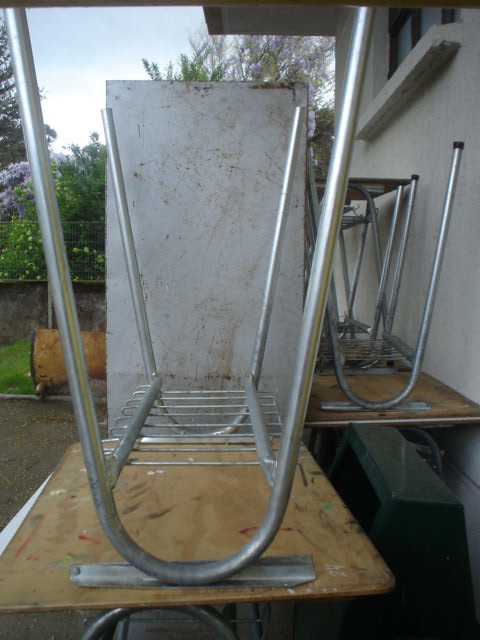The image depicts an outdoor area, likely part of someone's backyard, characterized by an evident lack of recent activity. In the center and bottom of the image, multiple tables are stacked surface-to-surface; the ones on the bottom are upright with metal U-shaped legs, while those on top are placed upside down. A notable detail includes a refrigerator barely visible from the side, marred by a brown liquid-like stain. Surrounding these tables are even more stacks, including one configuration where an upright table stands atop another upside-down table. In the upper right, the edge of a white building is visible, featuring a sleek windowsill and a black frame, partly shaded by an overhead structure. The background is filled with lush greenery, with a specific neighbor's green tree peeking through a black concrete fence topped with wire mesh. Yellow and white flowers contrast against the blue sky, providing a hint of vibrant life amidst the otherwise neglected scene.